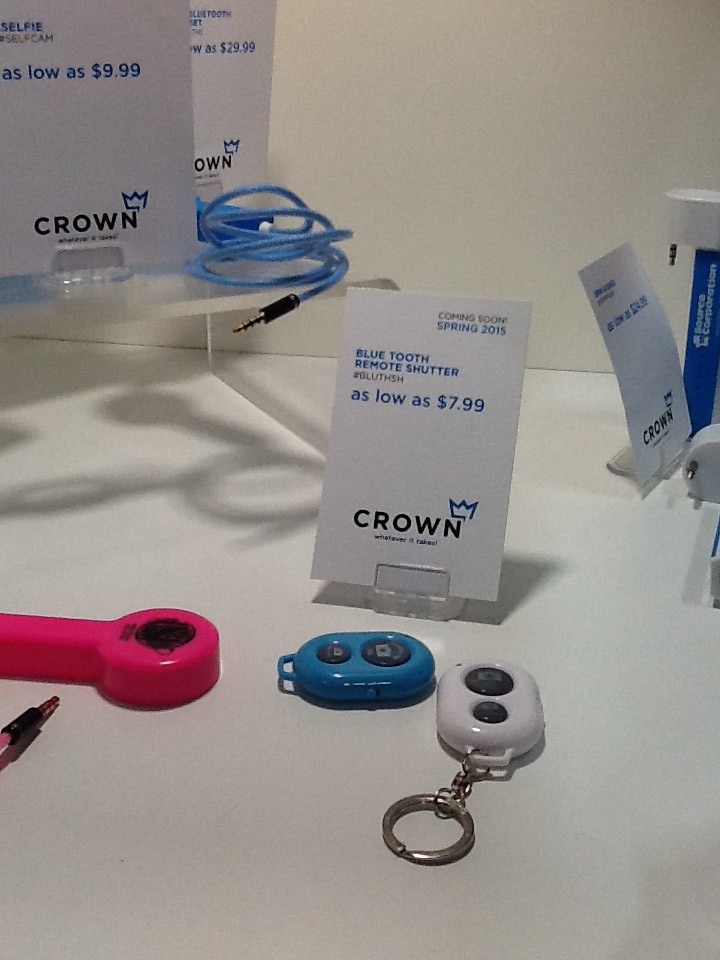In the center of the image stands a white card on a clear clip, announcing, "Coming Soon: Spring 2015, Bluetooth Remote Shutter, as low as $7.99." The card features the Krang logo, a blue crown above the letter 'N'. In front of the card, three remote shutter devices are displayed. On the left is a pink, elongated device with a single black circular button. In the middle is a blue, oval-shaped remote with two black buttons. The rightmost device is white, also with two black buttons, and it includes a silver keychain attached. Background elements include additional signs promoting related products with various prices and blue signage, reinforcing the Krang brand and its offerings.